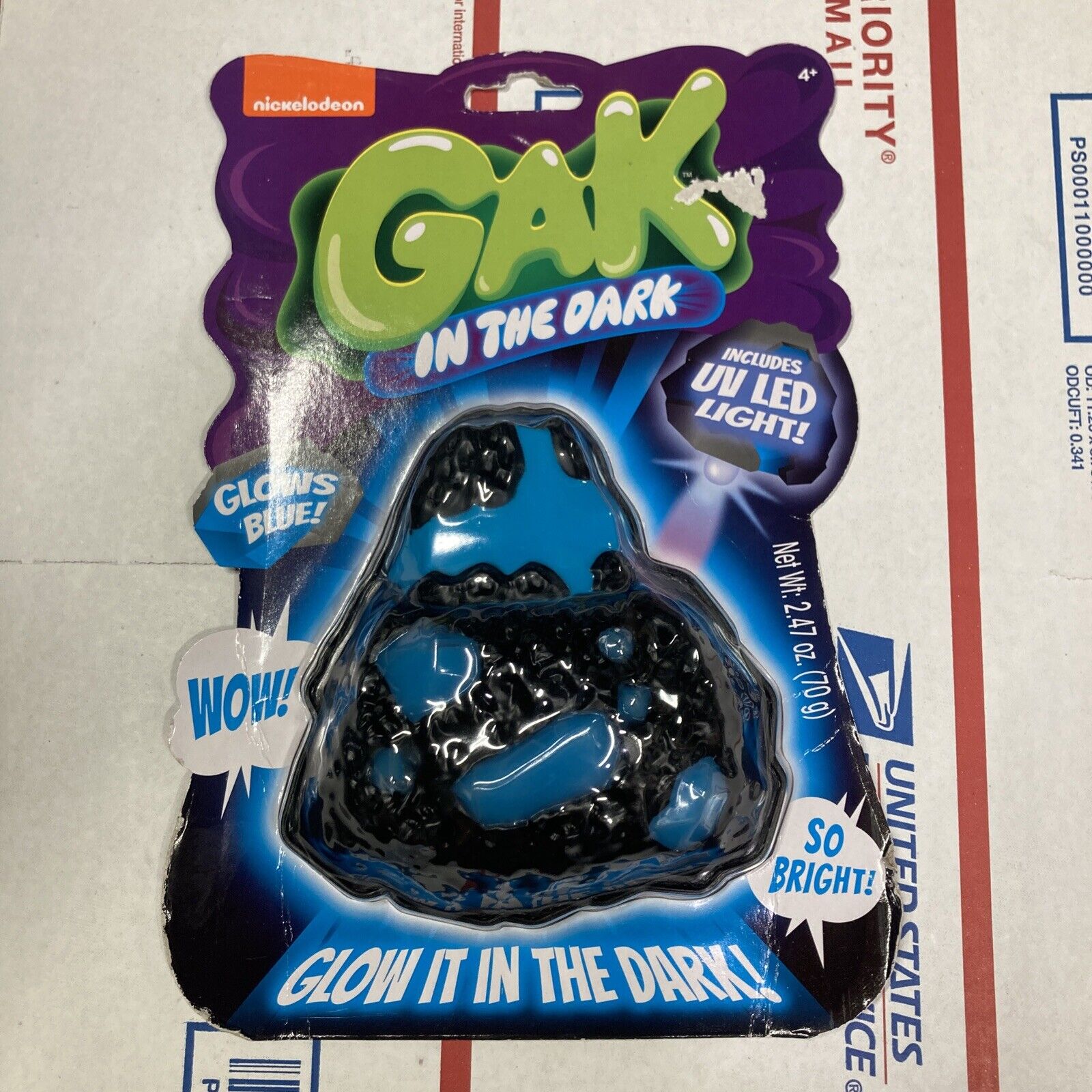The image depicts a vibrant, kid's toy called "Gak in the Dark," produced by Nickelodeon. This oozy, gunky blue slime glows brightly in the dark, thanks to its inclusion of a UV LED light. The toy is contained within a bubble blister pack that is unopened, displaying the product clearly. The packaging features prominent exclamations advertising its glow-in-the-dark capabilities and shows the word "GAK" in a striking pukey green color. The toy is set against a backdrop of a USPS delivery box, which is folded out flat, suggesting it was recently mailed. The overall design and bright colors of the packaging make it clear that this is an exciting, eye-catching present likely intended for children.